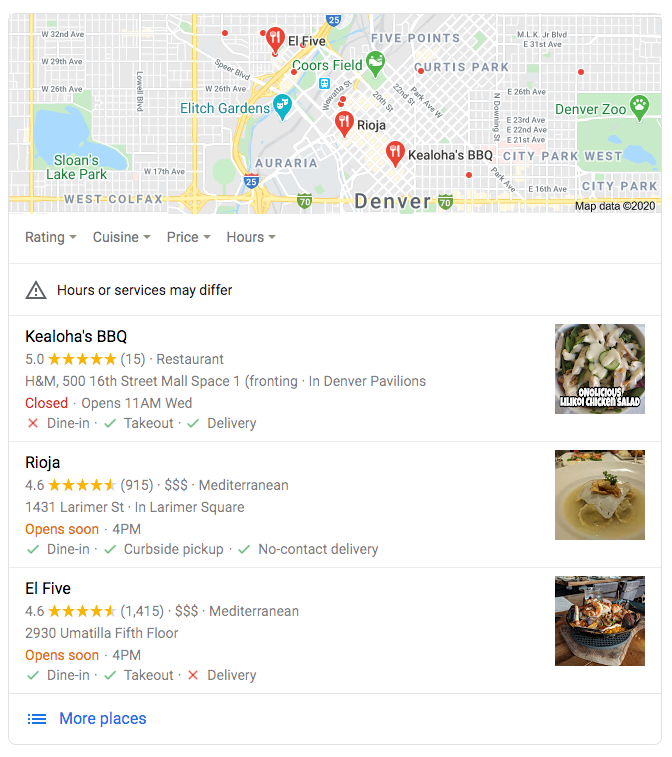Displayed on a map of Denver, Colorado, are three highlighted dining establishments, each represented by red dots indicating their locations. The first restaurant is Kealoha's BBQ, renowned for its delicious offerings and boasting a perfect 5-star rating across 15 reviews. This establishment offers takeout and delivery options but does not provide dine-in services.

The second featured restaurant is Rioja, a high-end Mediterranean eatery indicated by its three dollar signs suggesting an expensive dining experience. Rioja is highly acclaimed with 915 reviews averaging a 4.6-star rating. It offers dine-in, curbside pickup, and no-contact delivery options, catering to different dining preferences.

Lastly, L5, another Mediterranean restaurant marked similarly with three dollar signs, impresses with its upscale dining environment. This restaurant also enjoys a 4.6-star rating based on 1,415 reviews. It provides both dine-in and takeout services but does not offer delivery.

The map displays Denver's streets and the locations of these restaurants, offering a clear and detailed guide for food enthusiasts exploring the city's culinary landscape.